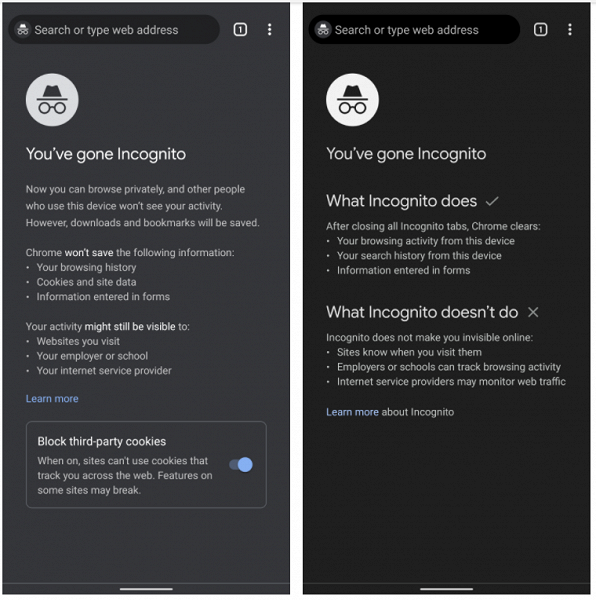Here's the cleaned-up and detailed caption:

"The image consists of two side-by-side screenshots taken from the Google Chrome browser on a mobile device, both displaying the Incognito mode interface. 

On the left, the screenshot shows an Incognito tab opened, characterized by the dark theme typical of this browsing mode. At the top left corner, there's a search bar featuring the Incognito logo with the text 'Search or type web address' inside. To the right of the search bar, there is a tab icon, followed by three vertical dots indicating the settings menu. Below these elements lies a prominent Incognito icon accompanied by text informing the user about the privacy features of Incognito mode. The text reads:
'You've gone incognito. Now you can browse privately, and other people who use this device won't see your activity. However, downloads and bookmarks will be saved. Chrome won't save the following information: your browsing history, cookies and site data, information entered in forms. Your activity might still be visible to websites you visit, your employer or school, your internet service provider.' Beneath this, there's a 'Learn more' link and a toggle switch labeled 'Block third-party cookies.' The switch is positioned next to an explanatory note: 'When on, sites can't use cookies that track you across the web. Features on some sites may break.'

On the right, the screenshot is nearly identical, showing another Incognito tab with the same layout and informational text. However, this version does not feature the 'Block third-party cookies' toggle switch at the bottom, indicating a slight variation in the interface or possibly an older version of the browser."